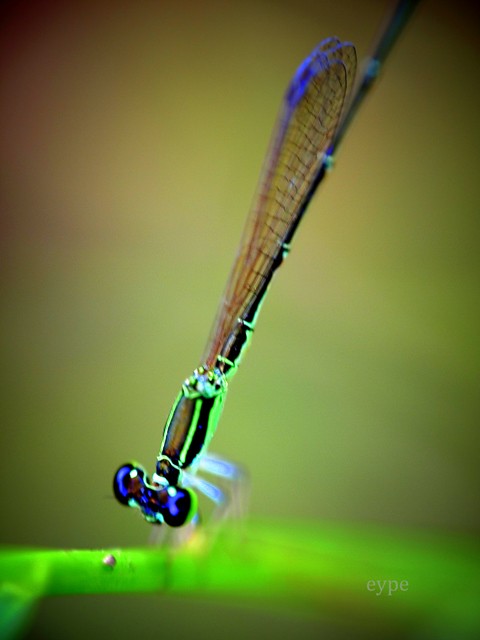This close-up image showcases a dragonfly perched on a green stem. The dragonfly's bright blue eyes are accentuated with neon green rims, facing towards the camera. Its slender body, primarily black with green stripes, extends upwards, ending in a finely tapered tail. Although the insect's six legs are somewhat blurred, the clear and detailed focus on its face and body highlights the contrast and vividness of its features. The wings, while closed, are mostly translucent with hints of brown and a subtle blue reflection under the light. The blurred background, predominantly green with touches of brown, indicates an outdoor setting amidst foliage, with some faint hints of orange and yellow, providing a natural camouflage for the delicate creature.